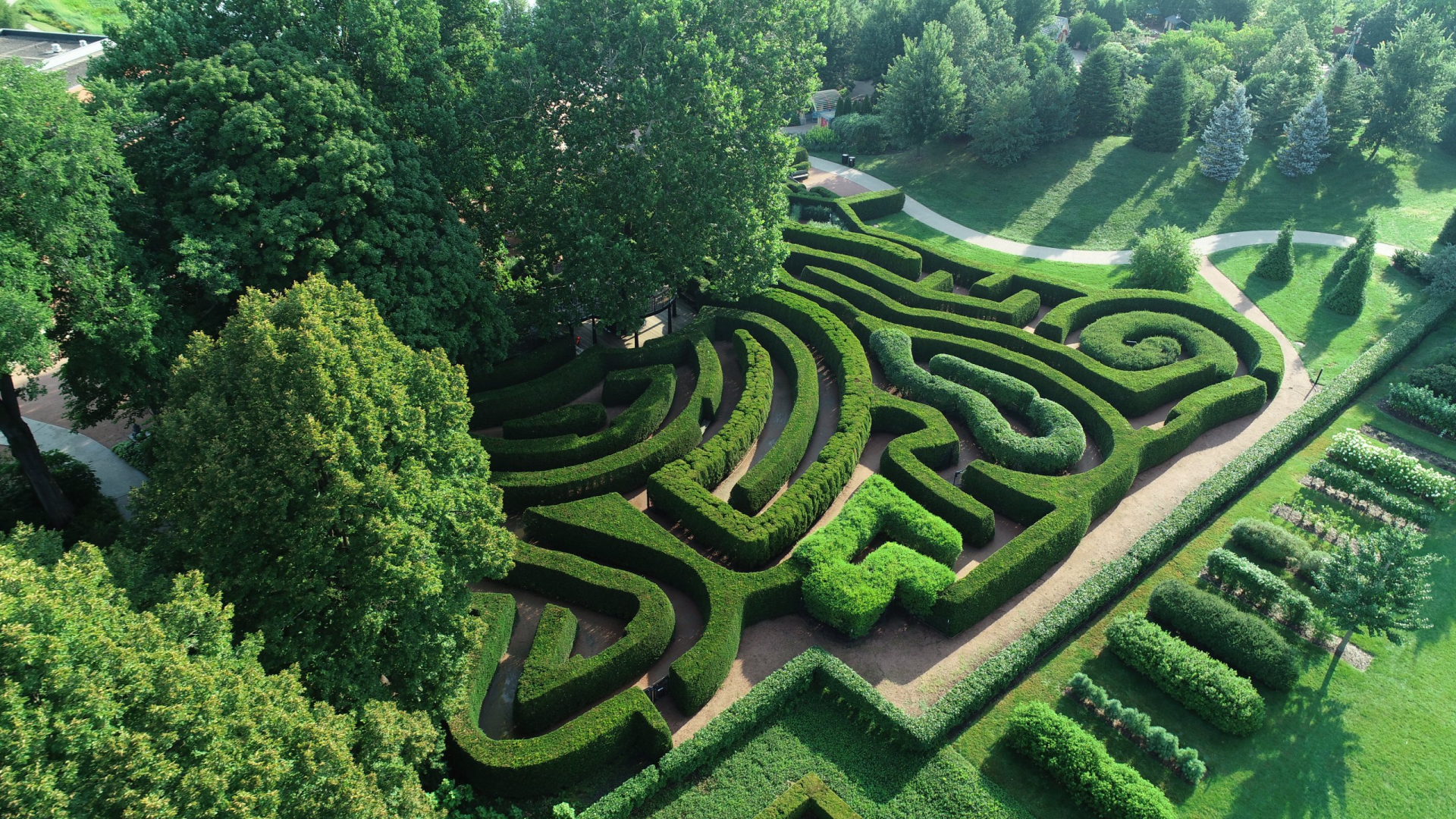The aerial photograph captures a meticulously designed garden within a large estate, showcasing a labyrinthine maze crafted from precisely trimmed hedges. Dominating the center of the image, the maze features intricate patterns, including spirals and long straight pathways, allowing visitors to meander through it while trying to find their way. The maze, composed of light and dark green shrubs, contrasts strikingly with the gray pathways winding through it. 

To the right of the maze, a well-manicured lawn is adorned with symmetrical rows of various types of shrubs and flower plants, bordered by angular, low hedges that run across the bottom right quadrant and make a strategic left jog. The top of the image reveals smaller, conical trees, while the left side is dense with larger, mature trees. Despite the vegetation partially obscuring parts of the maze, the lushness of the entire scene is evident. Surrounding the maze and integrating with the overall landscape is additional vegetation, including tree-lined areas and other garden elements, hinting at the expansive and grand nature of this estate's design.